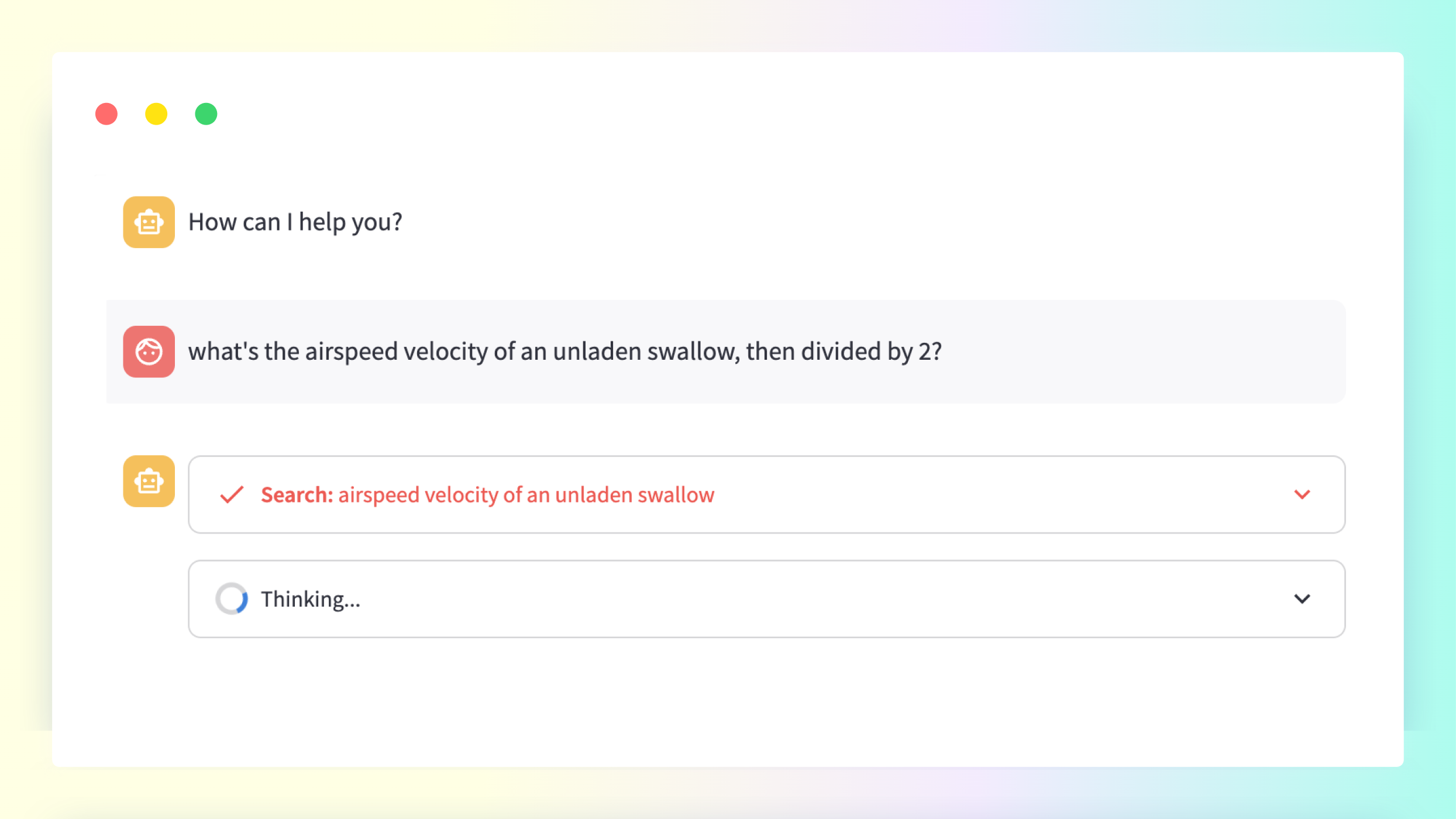The image depicts a user interface window, likely belonging to an Apple AI program such as Siri. The foreground showcases a text message box where a conversation is taking place. The topmost message is a prompt from the AI assistant asking, “How can I help you?” Below this, a user queries, “What’s the airspeed velocity of an unladen swallow divided by two?”

The AI assistant's response is captured mid-process. It displays a check-marked suggestion to “Search airspeed velocity of an unladen swallow,” followed by a thinking indicator, signifying that the AI is still processing the request. The main interaction box is predominantly white, creating a clean and minimalistic appearance.

The background behind this text box features a pastel sunburst gradient. It transitions from a creamy yellow, evocative of Easter-themed colors, to an oceanic, Caribbean teal hue on the right, adding a vibrant yet calming visual element to the overall design.